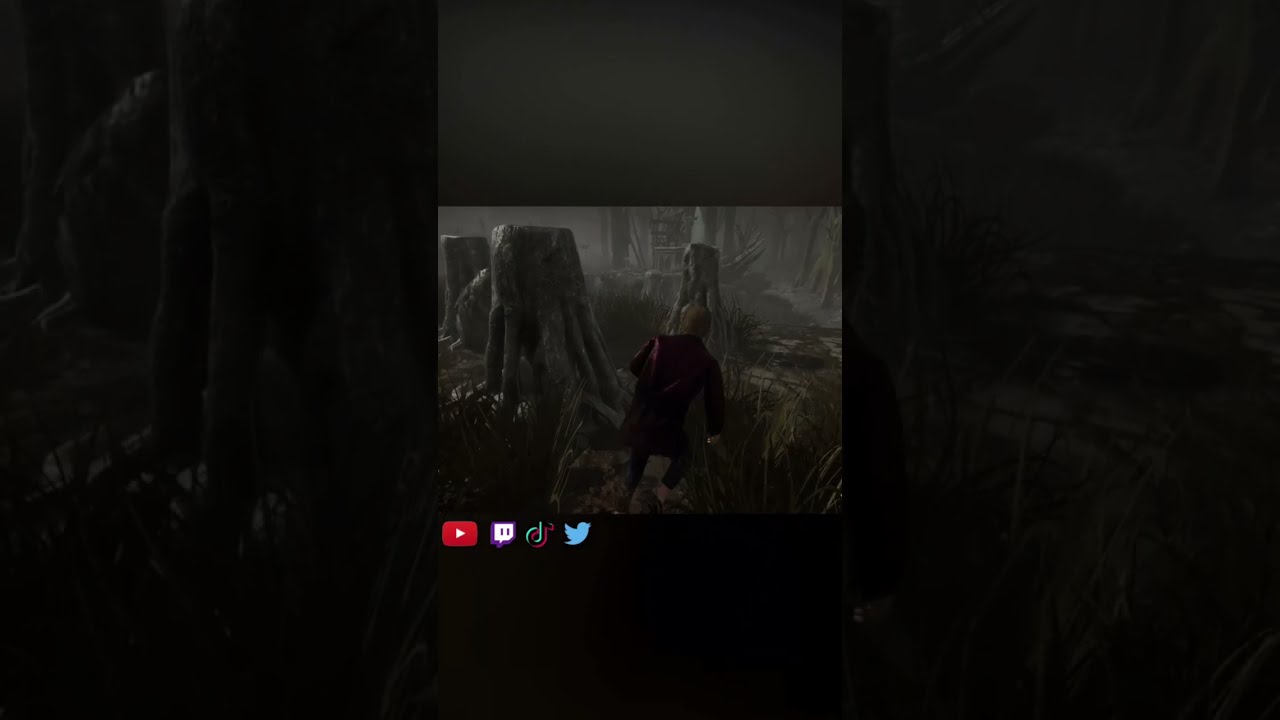This image appears to be a dark, foggy screenshot from a fantasy video game, showcasing a heavily wooded area with a male character moving away from the camera. The character, depicted in a maroon long-sleeved top and dark pants, may be barefoot or wearing light brown shoes and appears to have light-colored hair, possibly blond. The eerie forest features tall grasses, large tree trunks with their tops cut off and exposed roots jutting from the ground. In the background, more ominous trees and possibly parts of a wooden structure, like a house or a chest, are faintly visible. The visibility is poor due to the darkness and fog. The image is further complicated by being presented in a small central square surrounded by a dark border, which amplifies the overall gloom. Social media logos, including YouTube, Twitter, Twitch, and possibly Discord, are overlaid in the bottom left corner, suggesting this screenshot might be shared from the game on various platforms.